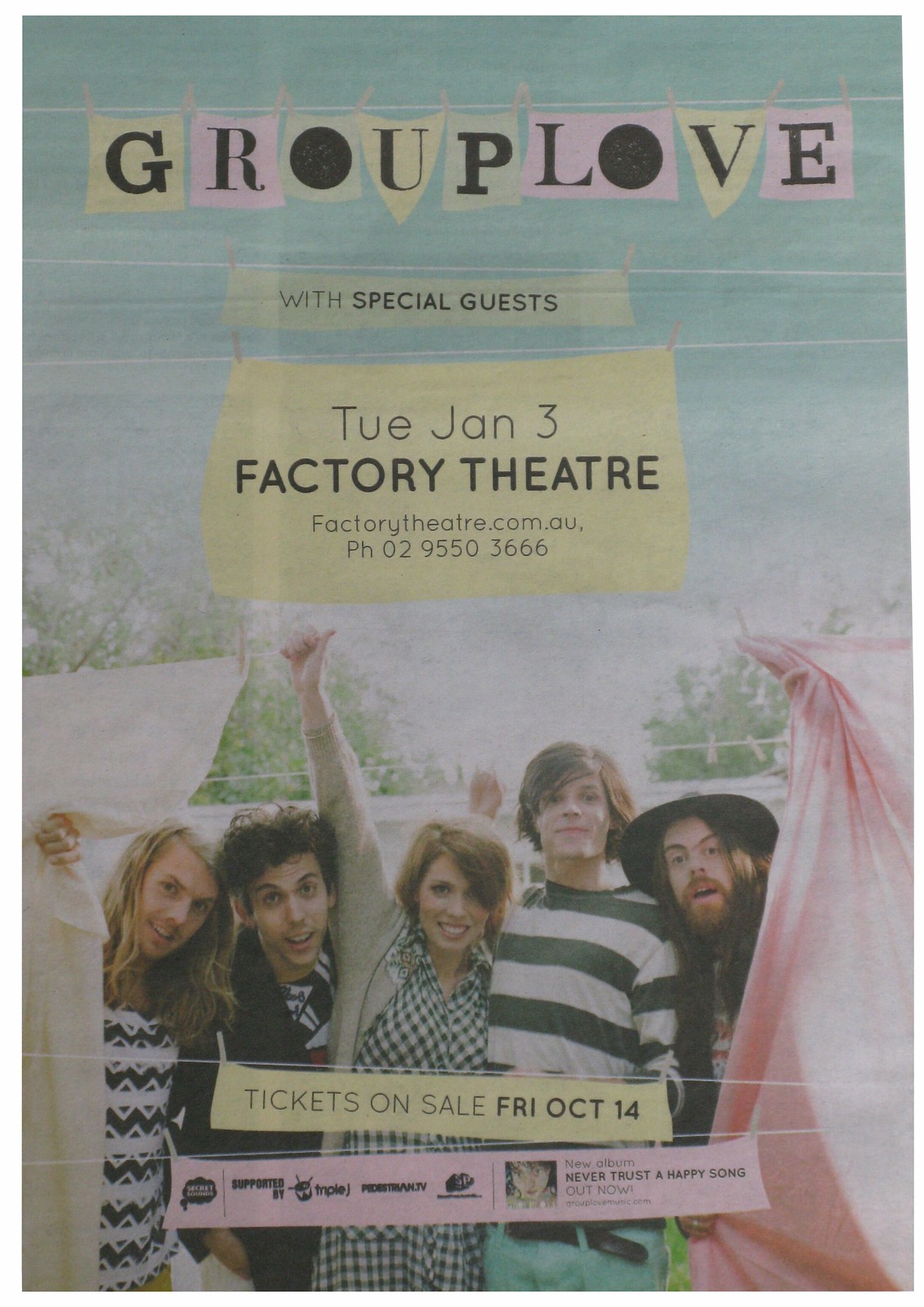This concert poster for the band Group Love, with their new album "Never Trust A Happy Song" out now, features the band prominently in the foreground. The image showcases the five band members: a man with long hair on the far left, a man with curly hair next to him, a woman in a green plaid dress, a man in a green and white striped shirt, and another man with long hair and a beard wearing a big hat. The background is decorated with letters on pieces of fabric pinned to a clothesline, spelling "Group Love" with each character individually styled in different colors and shapes. Beneath the band’s name, more fabric pieces announce "with special guests" and the event details: "Tuesday, January 3rd, Factory Theater, factorytheater.com.au, PH 02-9550-3666." Another clothesline display indicates that tickets go on sale Friday, October 14th. Additionally, sponsors and the album title are also mentioned, though the text is small and some specifics are difficult to read. The overall aesthetic captures a trendy, rock and roll vibe, complemented by the casual yet stylish appearance of the band members posing outdoors with a playful, quirky feel.